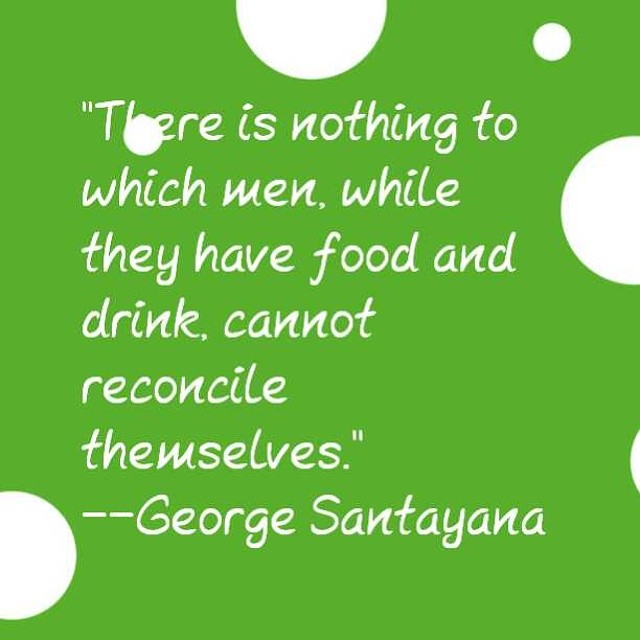The image is an inspirational poster with a lime green background punctuated by white polka dots. There are a total of six dots, some of which are partially cut off by the edges of the frame. The white dots are scattered: one at the top center, another at the bottom left, one on the right, two smaller ones on the center left and upper right, and a large dot obscuring part of the letter "H" in the text.

The quote reads, "There is nothing to which men, while they have food and drink, cannot reconcile themselves," in a mixed upper and lower case white italic or handwriting-style font. Beneath the quote, to the left, there are two dash marks followed by the name George Santayana. The text extends from the top center to the bottom center of the image, making it predominantly text-based.